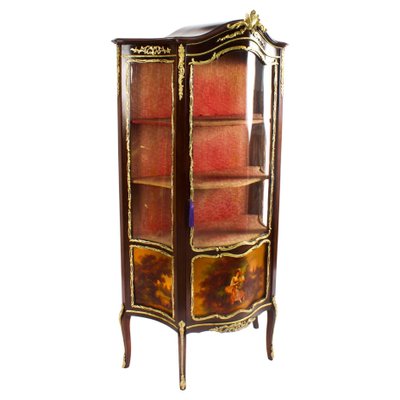The photo depicts a vintage, ornately designed black wood cabinet with gold trim and ornamentation. Standing on four wooden legs with gold accents, the cabinet features four distinct sections. The lower section is closed off and embellished with an image of a person on its front panel. The top three levels are enclosed in glass, allowing visibility of the empty shelves within, which are backed by a dark to light red wooden panel. The cabinet has an elegant, curved top adorned with a gold emblem. Photographed from a corner angle, the detail of the cabinet's craftsmanship and its potential use as a display case for items such as silverware or china is clearly visible.